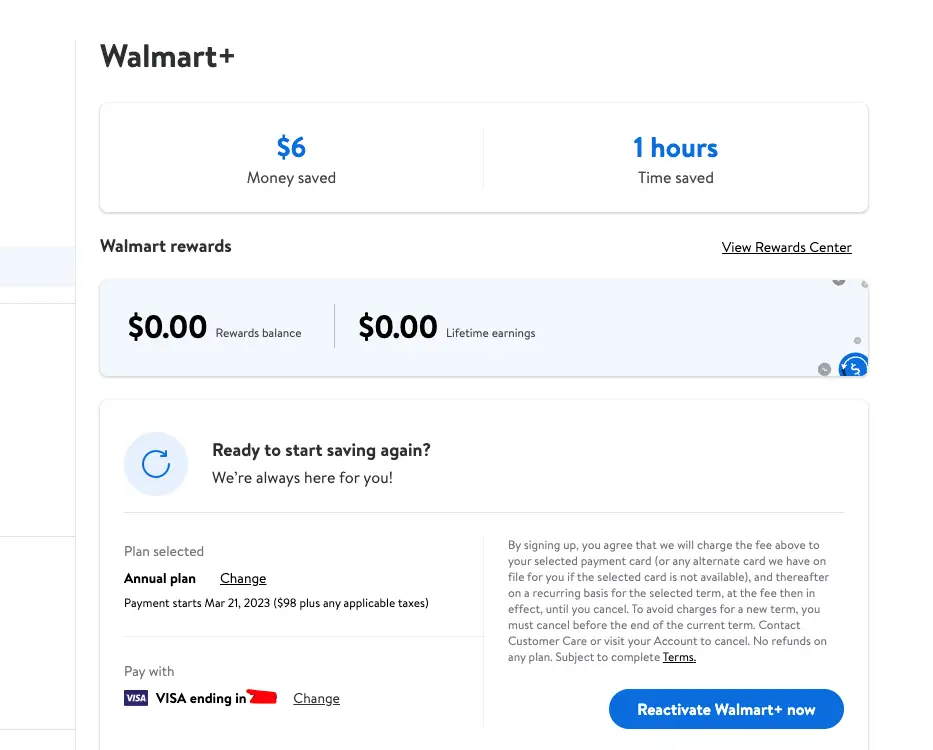The image is a screenshot of a Walmart Plus account dashboard. At the top, the title "Walmart Plus" is prominently displayed. Below this, within a box, it indicates a savings of $6 achieved in one hour, emphasizing the time saved. Following this, there's a section titled "Walmart Rewards," with an option to "View Rewards Center" on the right side. The dashboard further displays a reward balance of $0 and lifetime savings of $0. It prompts the user with "Ready to start saving again? We're always here for you."

Additionally, it shows that the selected plan is the annual plan with an option to "Change" the plan. Payment details indicate that a Visa card, with the ending digits obscured, is set for payments. On the left side, there's a note signifying agreement to terms upon signing up. At the bottom, a prominent blue button says "Reactivate Walmart Plus now."